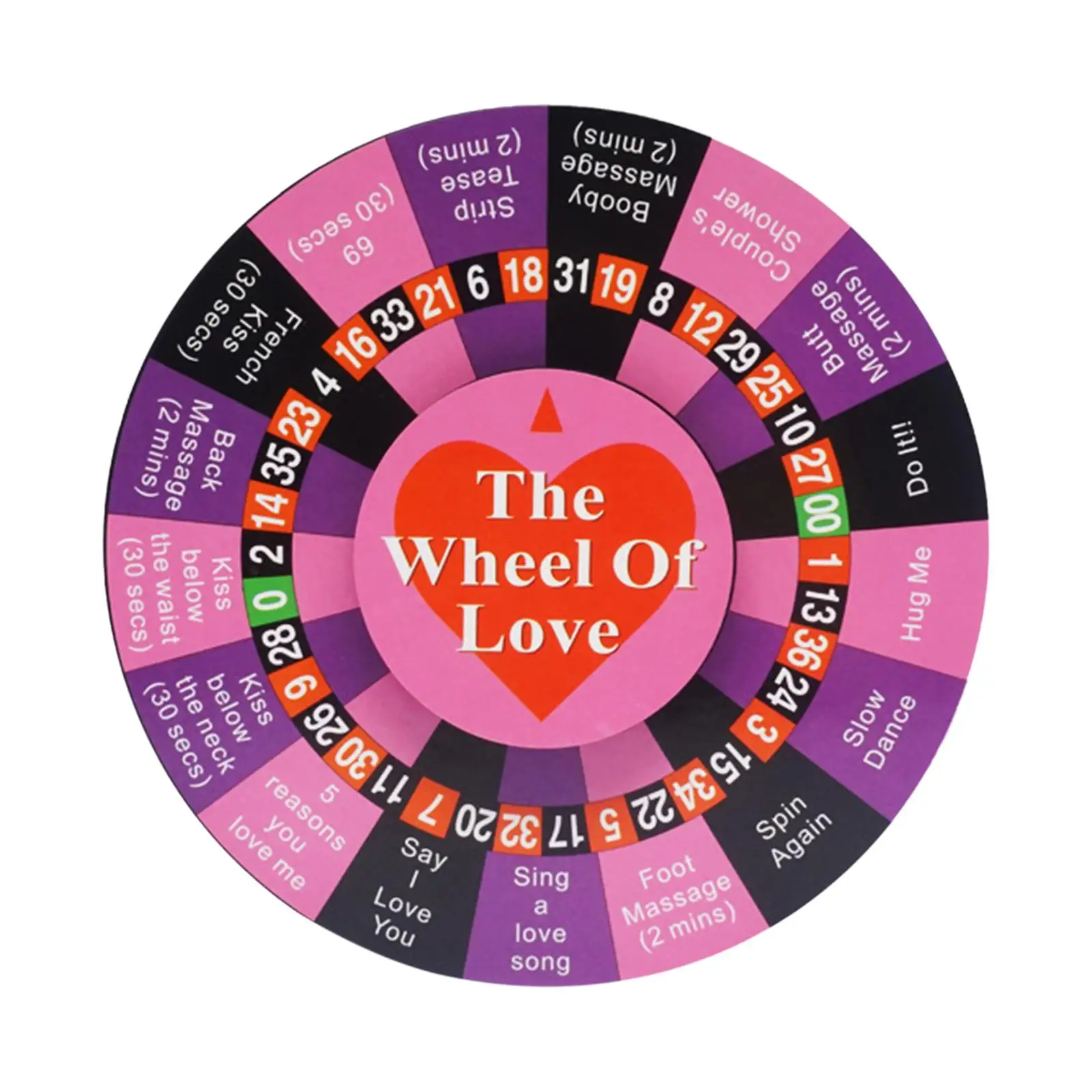The image features a meticulously detailed and vibrant roulette wheel against a plain white background. At the very center, a small circle approximately one inch in diameter sports a pink backdrop with a prominent red heart at its core. Above the heart, a small red triangle is placed, and the words "The Wheel of Love" are inscribed across the heart in bold white letters.

Surrounding the pink central circle, a series of small square shapes, each about half an inch tall, are arranged in alternating colors of black, pink, and purple. Enclosing these squares is another circle segmented into smaller squares with alternating black and red colors, featuring various numbers. Notably, two green squares on the left and right sides display the numbers 0 and 00, respectively.

Encircling this numerical layer, larger squares continue the alternating color scheme of black, pink, and purple, each bearing white text that proposes different romantic actions or questions. Examples of these prompts include:

- Kiss Below the Neck for 30 Seconds
- 5 Reasons You Love Me
- Say I Love You
- Sing a Love Song
- Foot Massage for 2 Minutes
- Spin Again
- Slow Dance
- Hug Me
- Do It
- 2 Minute Butt Massage
- Couple's Shower
- 2 Minute Boobie Massage
- 2 Minute Strip Tease
- 30 Seconds of a 69
- 30 Seconds of a French Kiss
- 2 Minutes of a Back Massage
- 30 Seconds of Kiss Below the Waist